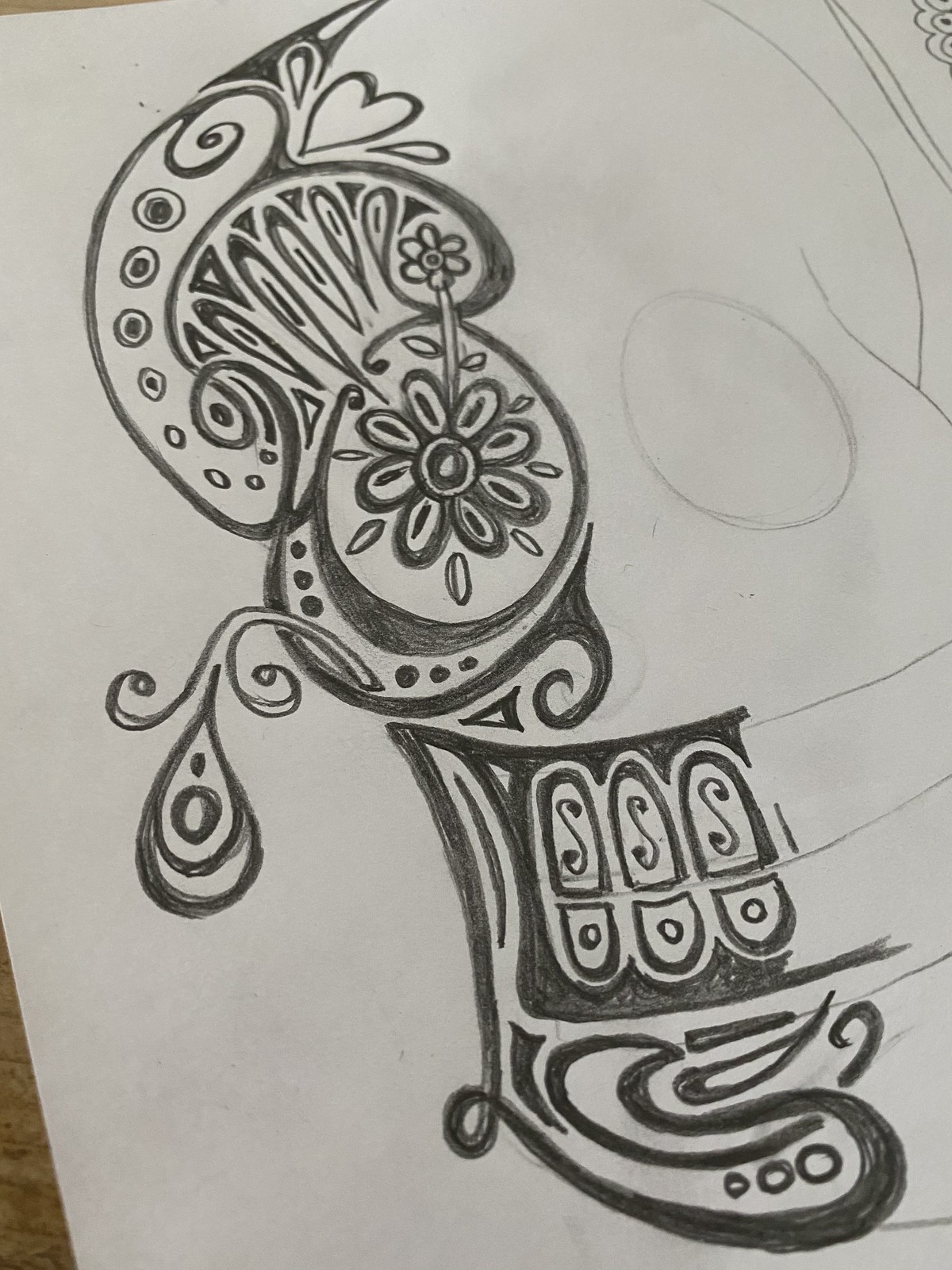This black and white pen-and-ink drawing on a beige piece of paper features a partially finished, abstract design that resembles a stylized skull, similar to those seen in Day of the Dead motifs. The right side of the drawing consists of a simple, lined outline of the skull's basic shape, including the eyes and mouth. Contrasting this, the left side is far more ornate and detailed. There, one eye is represented by a flower with petals and circles radiating from it, connected by ornate, dotted lines. The upper part of the design features L-shaped curved lines with small black circles, while below them, flower-patterned elements emerge from circular sections. The lower section of the skull showcases elongated ovals and intricate S-shaped forms within a rectangular structure with an arched top, which collectively evoke the appearance of a shoe print. The bottommost part of the design features a large swirling S shape. This composition combines geometric patterns and floral motifs, lending it the potential to be a unique tattoo design.